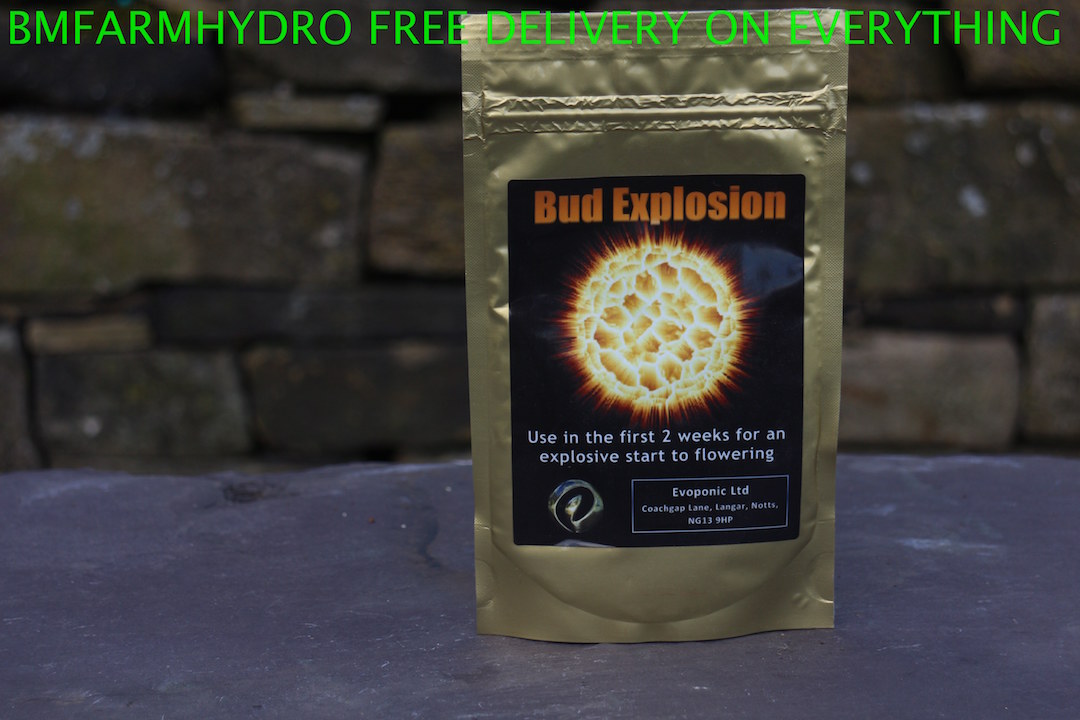The image depicts an advertisement for BM Farm Hydro, prominently featuring a resealable gold package with a black label branded "Bud Explosion." In bold neon green letters at the top, the ad announces "Free delivery on everything." The gold package, marked with an orange graphic of a bud exploding like the sun, is described as ideal for use in the first two weeks to promote an explosive start to flowering. Below the striking graphic, white text provides further product details, including its use instructions. The package sits on a smooth gray concrete surface in front of a background of neatly stacked brown bricks. The label also mentions Evoponic LCD and Coach Gap Lane, Langer, with a partial postal code N-G-1-3-N-H-P.